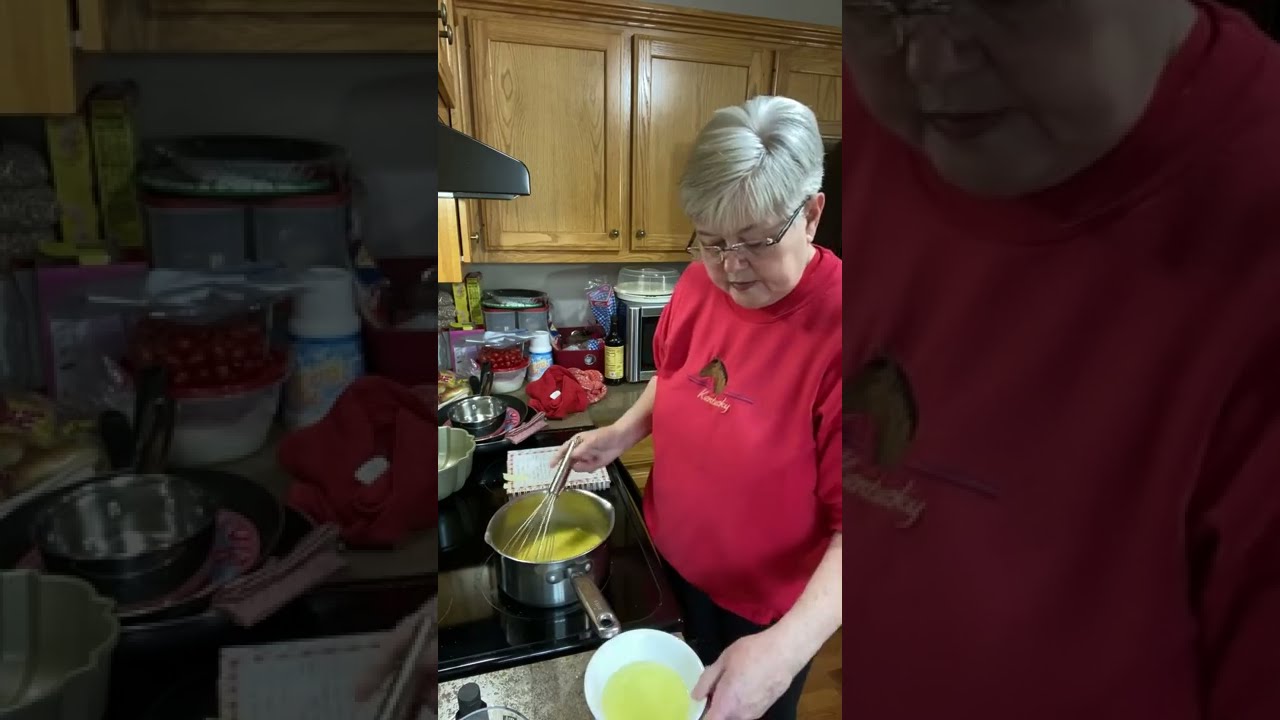The image captures an elderly, slightly overweight Caucasian woman with short white hair and glasses, deeply engrossed in cooking at her stovetop. She is wearing a distinctive red sweater with a small horse emblazoned on the chest. Positioned in her right hand is a whisk, actively stirring a yellow liquid—perhaps eggs or batter—in a silver pan. In her left hand, she holds a white bowl containing more of the yellow mixture. The background features a typical home kitchen with pale wooden cabinets, a microwave with its cover, and various kitchen items including a blender, spatulas, bowls, and a recipe book. A vent hood is visible above the black stovetop. The image appears to have borders on both sides, containing enlarged and faded segments of the central scene, creating a soft frame around her bustling kitchen activity.